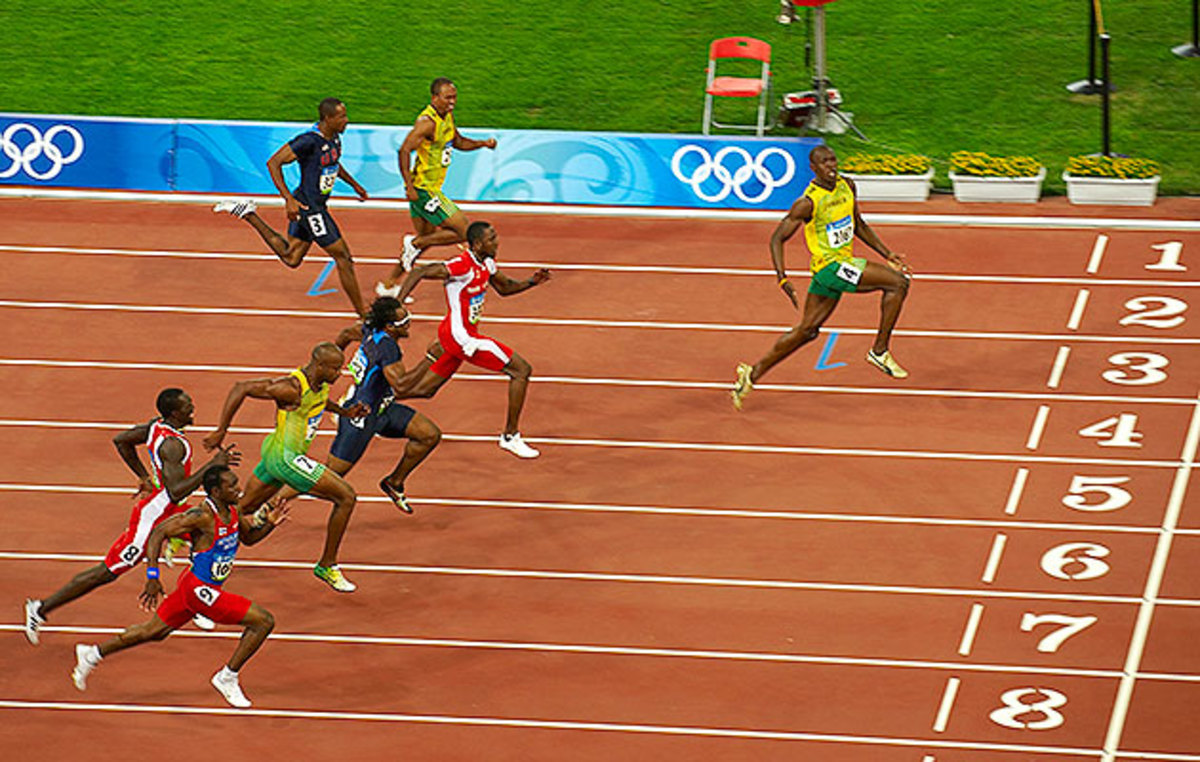This angled photo captures the intensity of an Olympic track race, showcasing eight African American runners in mid-stride. The athlete in lane four leads the pack, distinguished by his yellow top, green shorts, and white running shoes. His runner's bib, displaying the number 2367, marks his position as he surges ahead of the others. The track, a red clay dirt surface, is marked with numbered lanes, with the visible numbers 1 through 8 in the left corner. The runners, each adorned in various uniforms, highlight the diversity of competition: from red and white to dark blue with light blue trim, black, and red and blue combinations. 

In the backdrop, a blue banner with the iconic white Olympic rings underscores the event's prestige, set against meticulously manicured green grass. Notably, near the right corner of the track, three white rectangular pots with vivid yellow flowers add a touch of color to the scene. The athletes' dynamic motion is evident as they propel forward, with right legs thrusting into the air and hands poised by their sides, epitomizing athletic prowess.